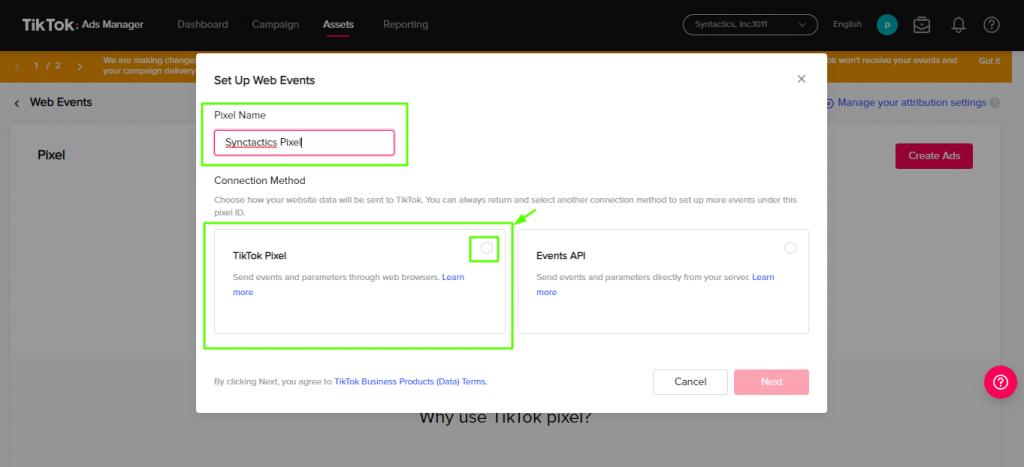The image depicts a screenshot of a TikTok page primarily displaying a black background with several tabs and icons on the right side. The entire page is overlaid with a gray tint, making it difficult to discern details and read the content clearly. Prominently visible are sections labeled "Web Events," "Pixel," and "Create Ads." An orange rectangular highlight is noticeable in the navigation area.

In the center, a white rectangular pop-up box is visible with an "X" button at the top right corner. The top left of this box states "Set Up Web Events." Within this pop-up, there is a text field labeled "Pixel Name," although the text within this field is blurry and difficult to read. Surrounding this area is a pink box with a green box enclosing it. Below this, a section labeled "Connection Method" is visible, accompanied by some unreadable text. Further down, there is additional text encased in a light green box with a green arrow pointing towards it, adding to the instructional aspect of the interface.